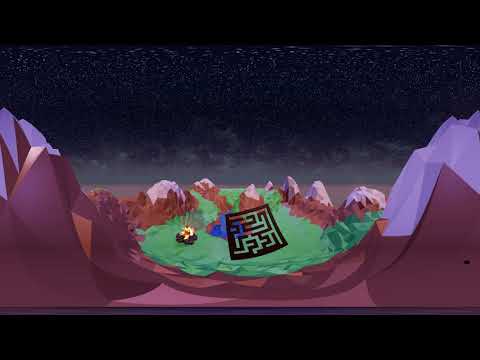The image portrays a 3D-rendered, video game-like scene with a distinct nighttime atmosphere. At the center of the image is a black square overlay with intricate lines resembling a maze, possibly hinting at a challenge or puzzle within the game world. This maze is superimposed on a valley nestled between two mountain ranges. The mountains on either side are characterized by their snow-capped peaks—represented by pixelated white tops—contrasting with their brown slopes. The valley itself features rolling green grass and a serene blue lake that extends further downward. Adding to the scene's detail, there is a round fire blazing on the left side of the valley. A single yellow flower can also be spotted amid the greenery. Above this lush landscape, the sky is depicted as a dark night sky filled with white dots symbolizing stars and clouds lying low on the horizon, all contributing to the serene yet intricate composition of the image.